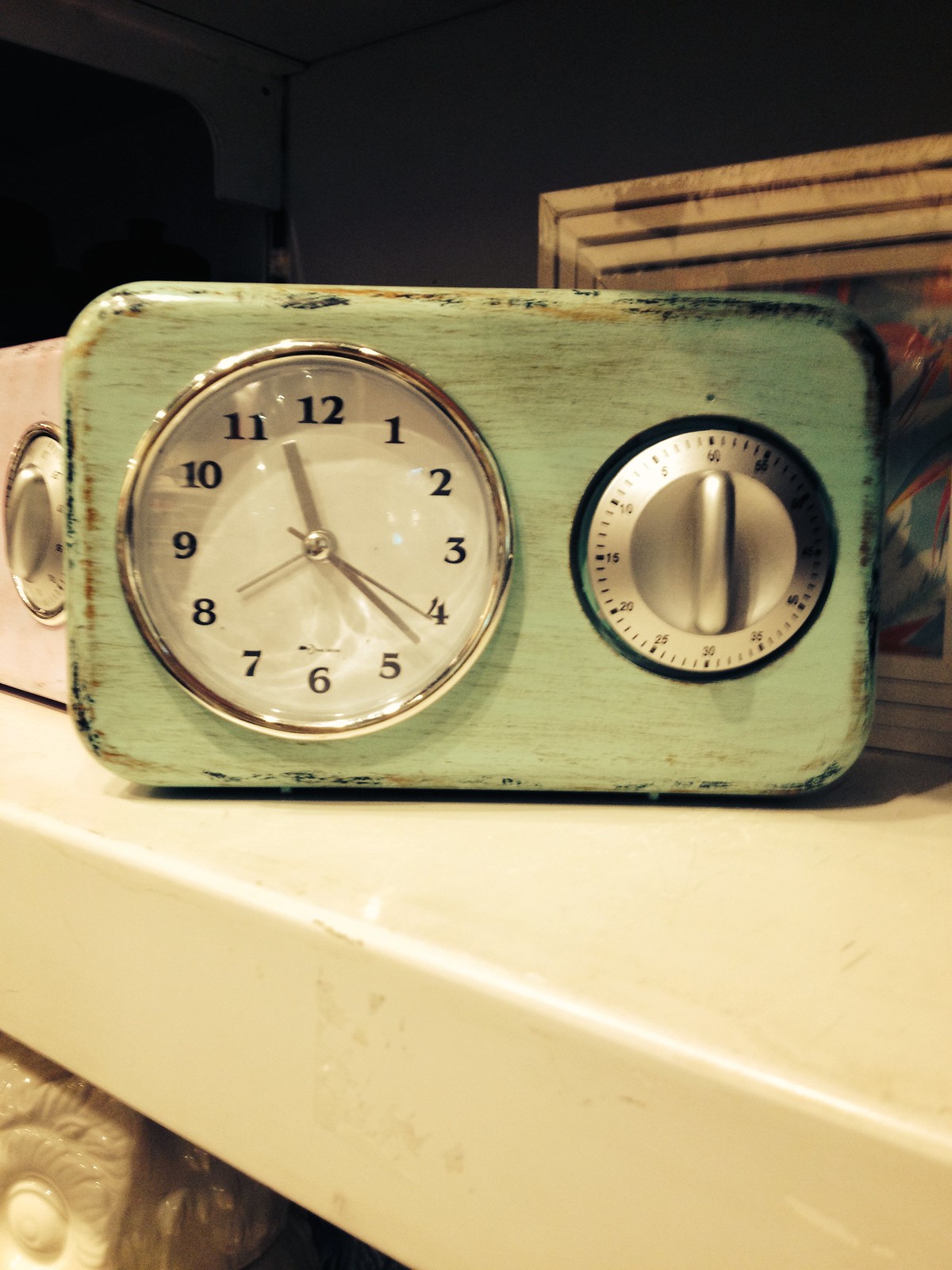This image features a weathered, mint-green kitchen clock with a built-in 60-minute timer. The clock, which exhibits a distressed finish with brown and black markings around its edges, is elegantly framed with a silver border. Its white face is adorned with black numbers ranging from 1 to 12, and the seconds, hours, and minutes hands are all silver. The timer, situated on the right-hand side of the clock, features a silver dial with increments marked from 5 to 60. The setup rests on a thick, white countertop, approximately 7 to 8 inches in thickness. Below the counter, a white porcelain item can be partially seen. Behind the clock, there is a wooden wall art or painting that has blue, red, and white decorative design elements. The overall background appears somewhat dark, and the upper section of the image reveals a white wall.